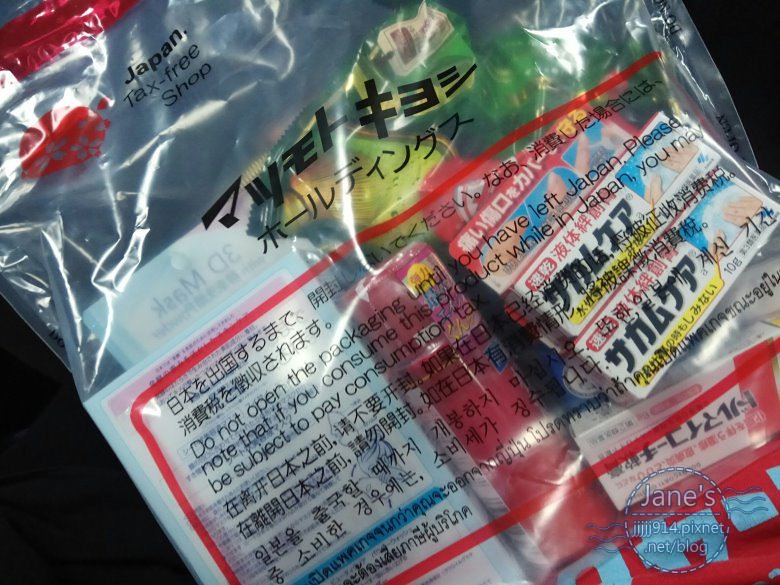The image captures a semi-transparent plastic bag containing various unidentified items, presumed to be packaging for products like pills or similar small goods. The bag features text in both English and Japanese, indicating it was purchased from a "Japan tax-free shop." Additionally, the label instructs not to open the packaging until leaving Japan to avoid consumption tax, and a notice in the bottom right includes a URL: jeans jjjjj914.pixnet.net/blog.